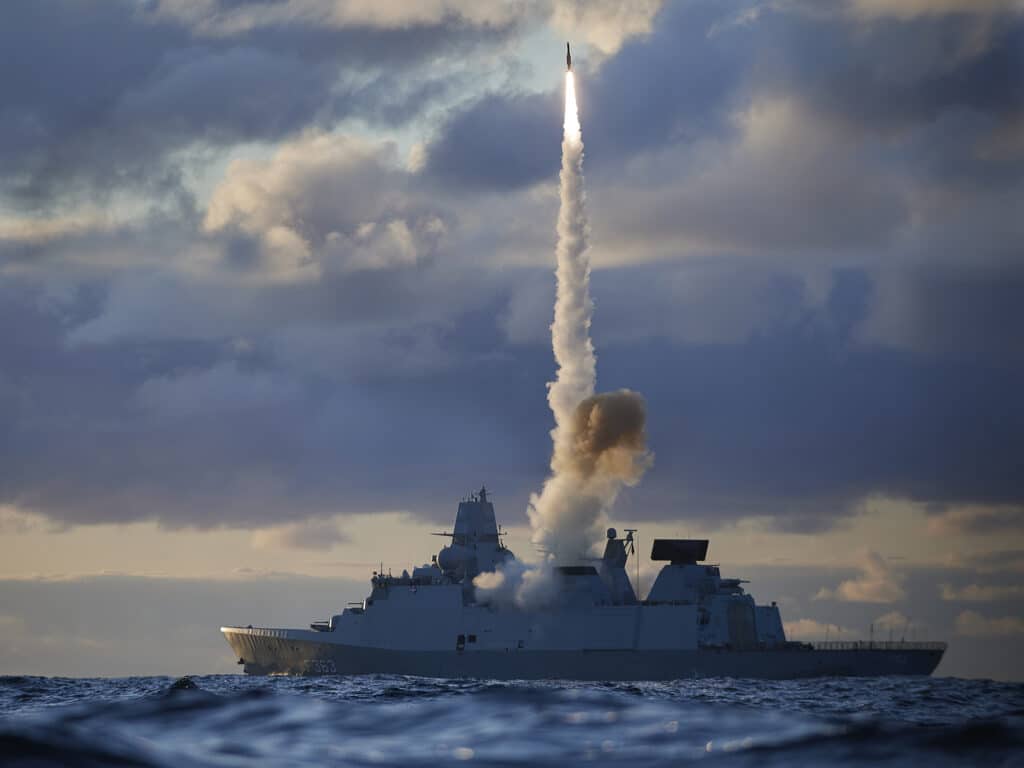The image depicts a gray or white guided-missile cruiser, possibly a foreign naval vessel distinct due to its "F-363" hull number, navigating choppy waters, likely in a sea or ocean. The ship, centered but positioned lower in the frame, features a helicopter deck at the back and appears to be part of a littoral combat system designed with an integrated forecastle. A missile, launched using a vertical launch system, soars high into the partially clear, overcast sky, which is filled with thick, white smoke and a trail of bright yellow-orange fire from the missile's tail. The reflection of sunlight suggests that it is either early morning or late evening, with the sun shining from the left side of the image. The ship and the dramatic plume of smoke and gases create a striking contrast against the dark, blue water and the cloud-filled sky.